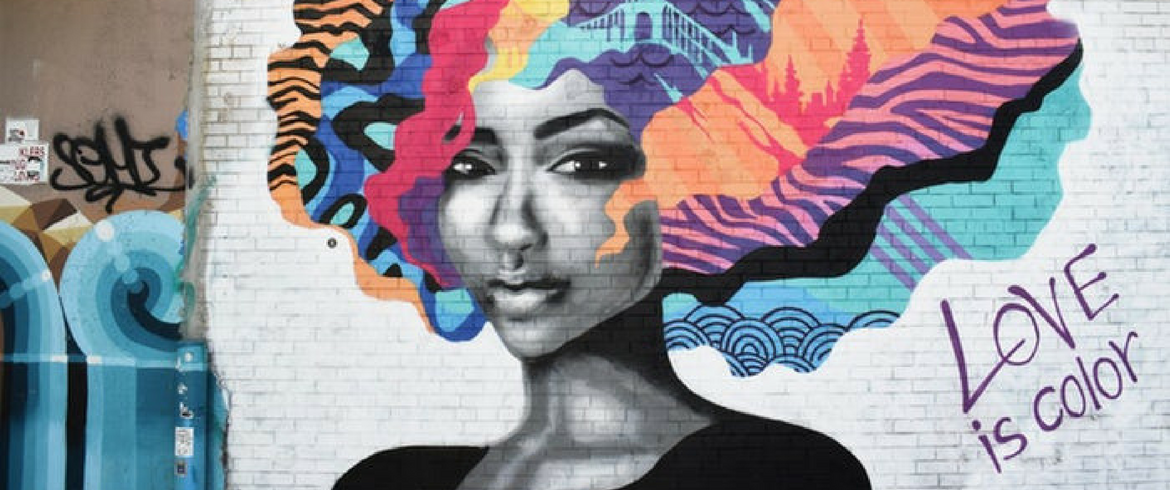The photograph showcases a vibrant mural painted on a white brick wall, depicting a woman with dark skin who appears to be African American. She is wearing a black top and is mostly rendered in black and white, except for her elaborate, flowing hair, which erupts in a kaleidoscope of colors and patterns. Her hair, styled in an afro, spills upward and outward in a series of striking sections. These sections include a vivid purple and pink zebra stripe, an orange and red area featuring tree-like shapes, and a dark purple and blue section highlighting a suspension bridge. Additionally, there are tiger stripes, blue spotted leopard patterns, magenta areas, and little blue spirals that add to the intricate collage. In total, there are about eight or nine distinct sections, each uniquely colored and patterned. On the bottom right of the mural, the phrase "Love is color" is written in purple text. The mural might be commissioned artwork, though it has a graffiti-like aesthetic.